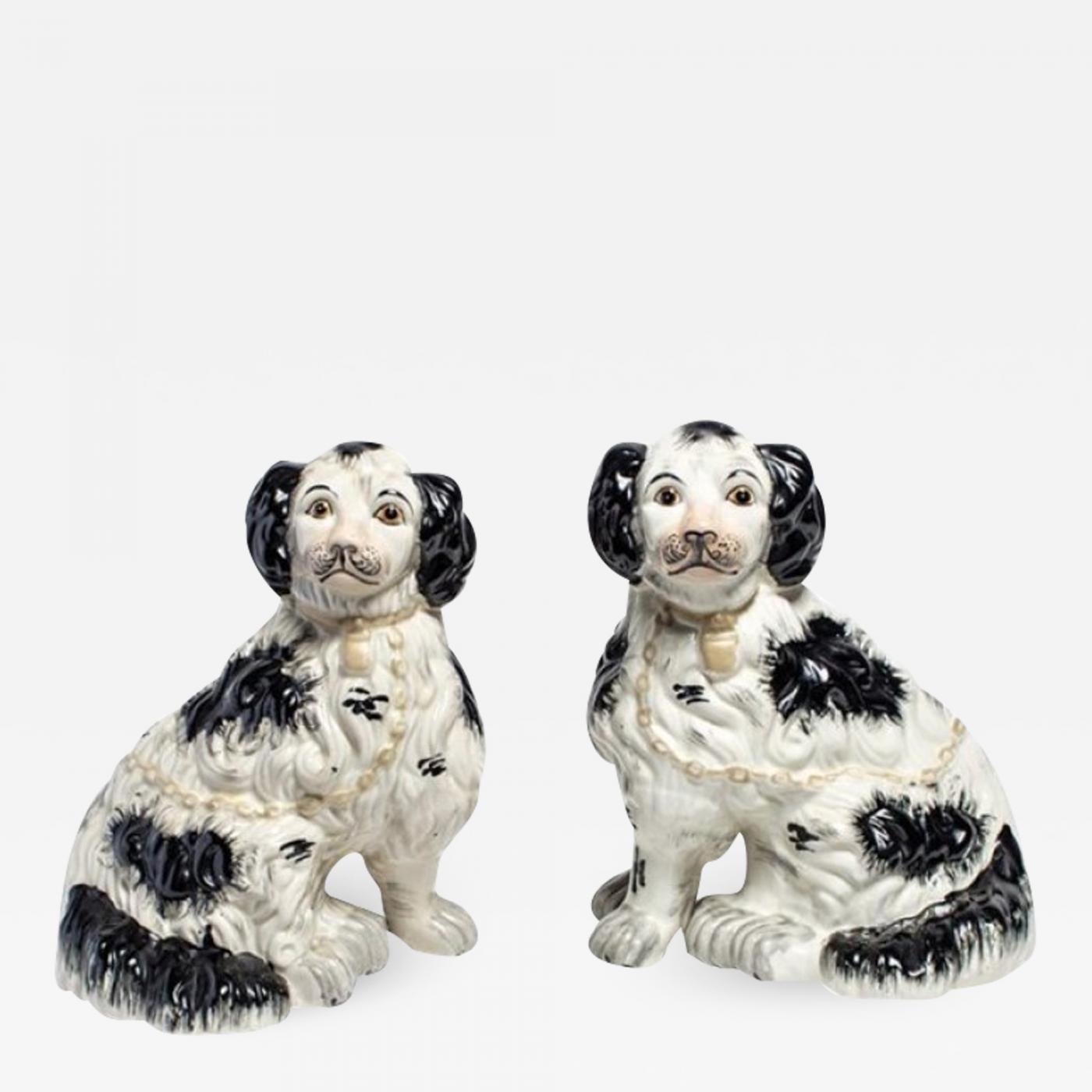This image displays two exquisite porcelain figurines, resembling a hybrid between dogs and cats with distinct human-like features. Each figurine is poised as a mirror image of the other, their bodies oriented sideways with their faces gazing directly forward. The animals are primarily white with black splotches, reminiscent of a cow print. Their ears are notably bushy and black, while their faces exhibit a peculiar mix of animal and human traits, including pronounced eyebrows and facial hair under their noses, resembling small mustaches. The eyes are undeniably human-like, contributing to their slightly startled and concerned expressions.

Both figurines are adorned with gold collars and chains, emphasizing their antique or potentially vintage origin and adding a touch of ornate elegance. The figures boast intricate details, such as a delicate black nose set within pinkish mouth areas. These details, combined with their stylized black tails and large, fluffy ears, underscore the hand-painted craftsmanship that differentiates each figurine ever so slightly.

With no visible background elements to provide context, the stark white backdrop isolates these unique and artistically ambiguous decorations, suggesting they could be part of a display, perhaps for sale, or simply a cherished piece of home decor. The figures stand out as elaborate, fantastical art pieces that seamlessly blend elements of various animals and human-like characteristics.